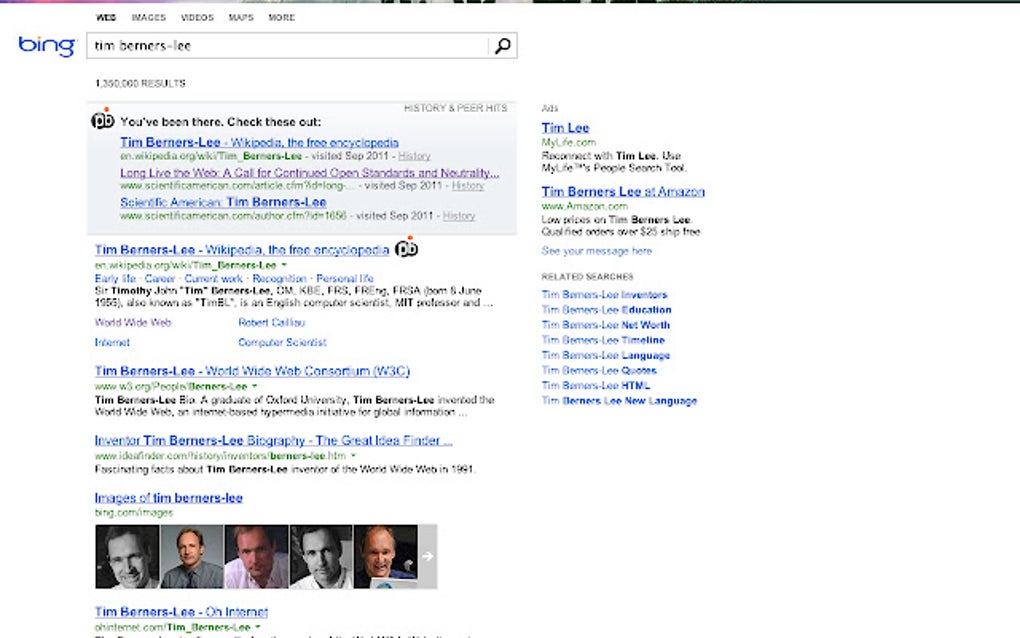The image displays a search engine results page for "Tim Berners-Lee." On the left-hand side, the background is white with the word "Bing" written in blue, featuring an orange dot on the "i." The word "Web" appears in bold black text, indicating this is the active page tab among options like Images, Videos, and Maps. Below these options is a search box with a white interior and a grey border, containing the query "Tim Berners-Lee."

The search results indicate about 1,200,000 hits. The top result appears to be an advertisement or highlighted suggestion, stating "You've been here, check this out," associated with a history-related topic, featuring terms like "history" and "peer hits."

The first few search results include:
1. "Tim Berners-Lee" from Wikipedia, labeled as "the free encyclopedia" in blue.
2. "Long Live the Web: A Call for Continued Open Standards" from Scientific American, also associated with Tim Berners-Lee, displayed in blue and purple.
3. "Tim Berners-Lee" Wikipedia entry again.
4. "Tim Berners-Lee" from the World Wide Web Consortium.
5. A blue link titled "Invested Tim Berners-Lee Biography, The Great Idea Finder."

Additionally, there are five images of Tim Berners-Lee shown towards the end of the results, presumably small thumbnail portraits of the individual.